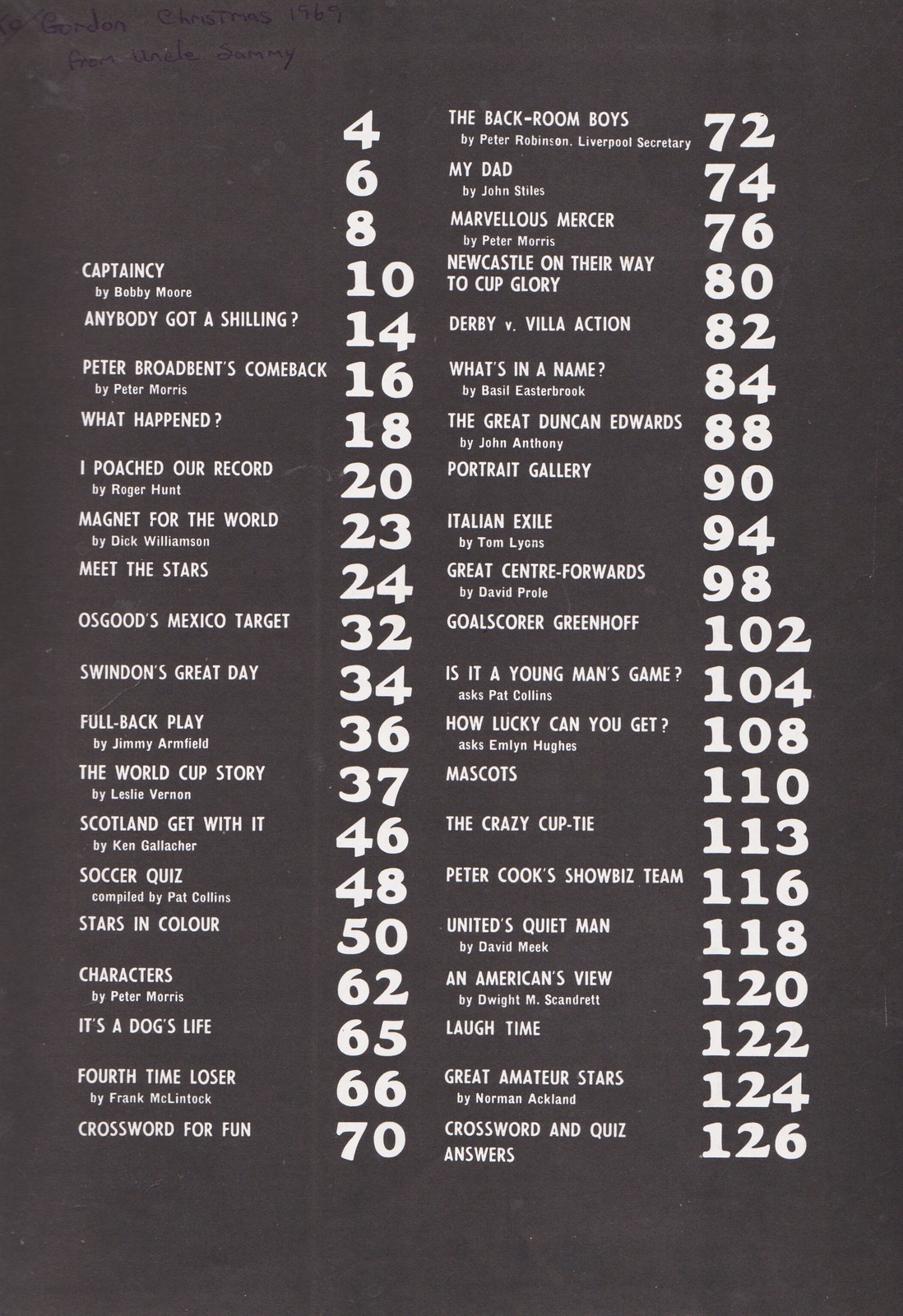The image displays a detailed list in a vertical, rectangular format with a black background and white text. It appears to be a content index possibly from a magazine or journal, featuring articles with titles and their corresponding page numbers. The first column on the left starts at the top with the number 4, followed sequentially by increasing numbers. Here are the titles and page numbers from the left column: 

- Captain C by Bobby Moore (10)
- Anybody Got a Shilling? (14)
- Peter Braw Bent's Comeback by Peter Morris (16)
- What Happened (18)
- I Post Our Record by Roger Hunt (20)
- Magnet for the World by Dick Williamson (23)
- Meet the Stars (24)
- Osgoode's Mexico Target (32)
- Swindon's Great Day (34)
- Fullback Play by Jimmy Armfield (36)
- The World Cup Story by Leslie Vernon (37)
- Scotland Get With It by Ken Gallagher (46)
- Super Quiz compiled by Pat Collins (48)
- Stars in Color (50)
- Characters by Peter Morris (62)
- It’s a Dog’s Life (65)
- Fourth Time Loser by Frank McClintock (66)
- Crosswords for Fun (70)

The second column on the right lists more titles and page numbers in a similar format:

- The Backroom Boys by Peter Robinson, Liverpool Secretary (72)
- My Dad by John Stiles (74)
- Marvelous Mercer by Peter Morris (76)
- Newcastle on Their Way to Cup Glory (80)
- Derby vs. Villa Action (82)
- What’s in a Name by Basil Easterbrook (84)
- The Great Duncan Edwards by John Anthony (88)
- Portrait Gallery (90)
- Italian Exile by Tom Lyons (94)
- Great Central Forest by David Prohl (98)
- Gold Squirrel Greenhoff (102)
- Is it a Young Man’s Game? Ask Pat Collins (104)
- How Lucky Can You Get? Ask Emily Hughes (108)
- Mascots (110)
- The Crazy Cup Tie (113)
- Peter Cook’s Showbiz Team (116)
- United’s Quiet Man by David Meck (118)
- An American’s View by Dwight Scanbritt (120)
- Laugh Time (122)
- Great Amateur Stars by Norman Ackland (124)
- Quiz Answers (126)

The numbers are listed in an almost sequential order, often increasing by twos, sometimes by one. The list starts with the number 4 and concludes with 126 in the second column. The titles include both specific articles and general features, some written by notable contributors.